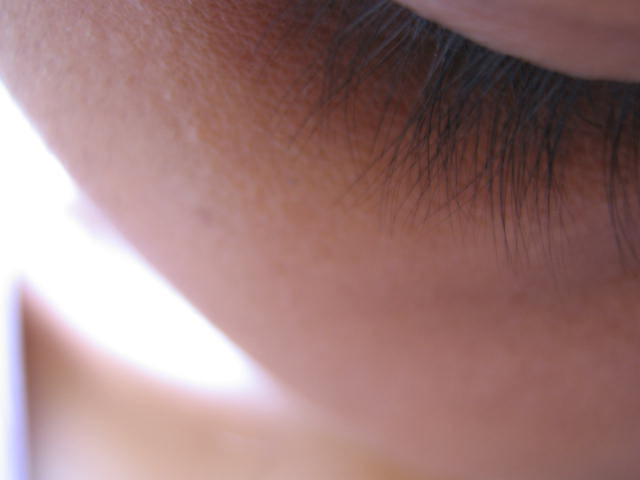This image is an extreme close-up of a person's face, focused primarily on their closed eyelids and eyelashes. The individual has smooth, Caucasian-type skin, and their thin, black eyelashes are densely packed. Some of the lashes are tangled, while others are straight. The photograph appears to be backlit, with a noticeable white glare emanating from the bottom left-hand corner, rendering that section of the image blurry. The main focal point remains the eyelashes against the eyelid. Although the extreme close-up might momentarily confuse the viewer about the nature of the subject, the prominent eyelashes indicate that it is indeed an image of a person's eye area with closed eyelids.